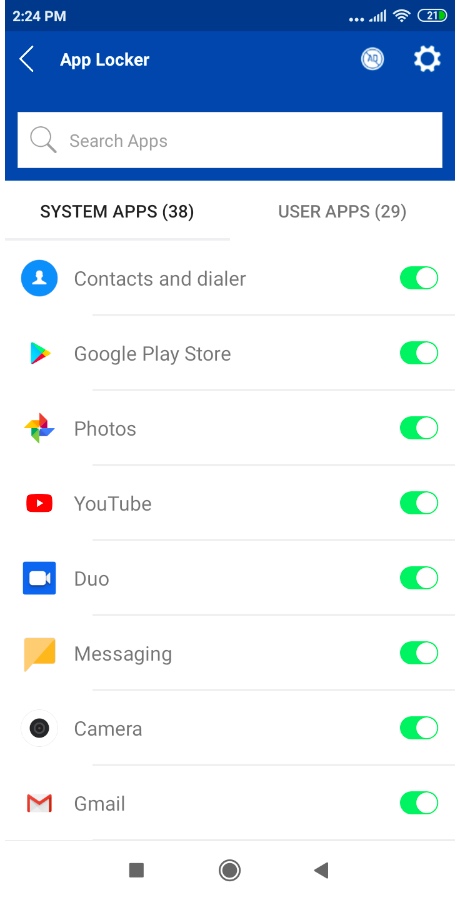The image displays the AppLocker interface on a smartphone, showcasing the system and user apps that can be locked. The screen is divided into two sections: system apps and user apps. Under the system apps section, several applications are listed, including Contacts, Dialer, Google Play Store, Photos, YouTube, Duo, Messaging, Camera, and Gmail. Each app features a toggle switch set to the "on" position in green, indicating that these apps are locked. 

The phone’s status bar is visible at the top, showing the time as 2:24 PM, a battery level at 21%, and standard Android navigation buttons (square, circle, triangle) at the bottom. The interface also includes a search function for finding specific apps within AppLocker and an "ad-free" icon located in the top right corner. This image appears to be demonstrating the use of AppLocker for securing various applications on the device.